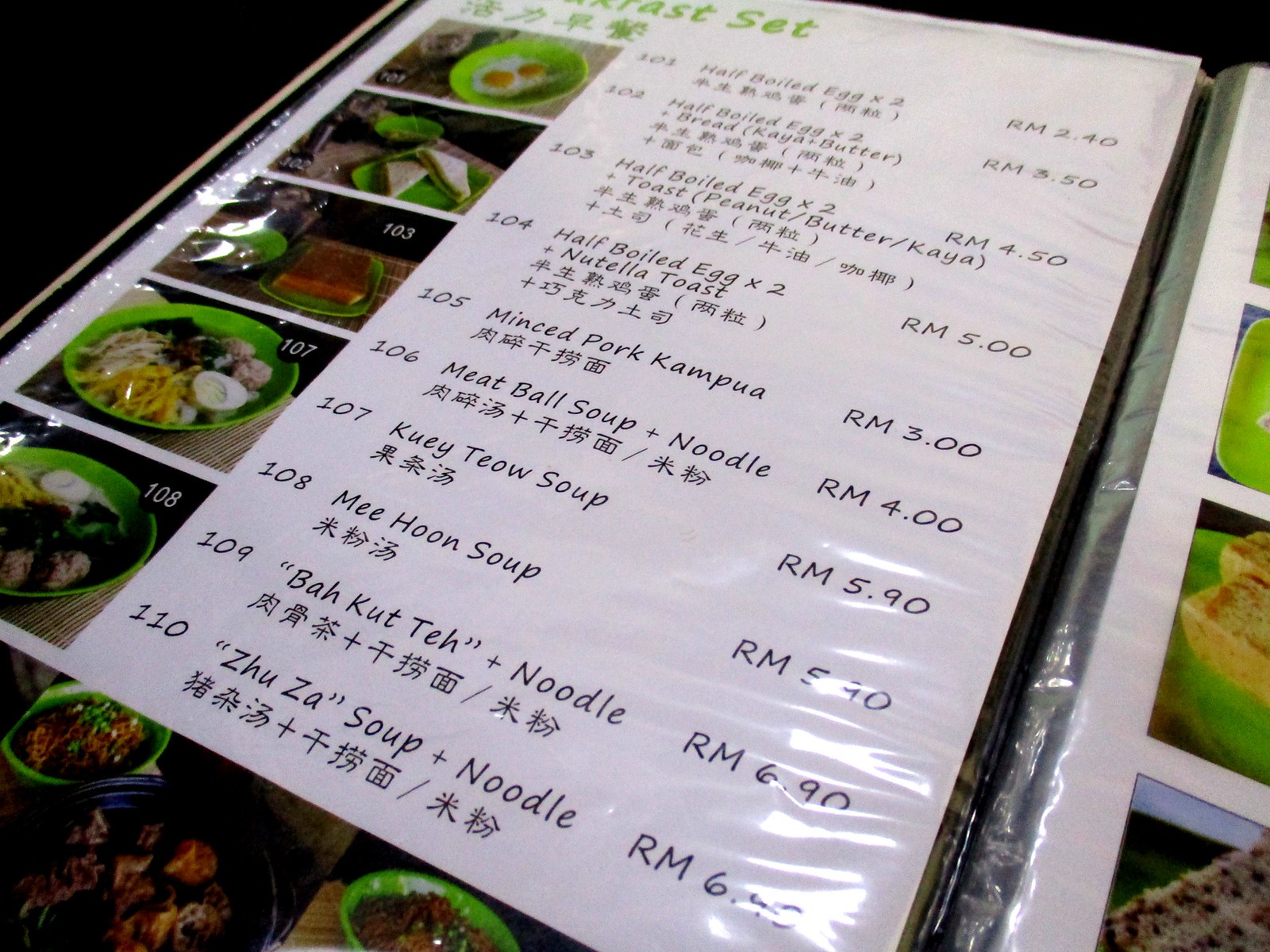This image depicts a laminated menu page from an Asian restaurant. The layout features a white background with a vertical column of five dish images on the left side. Each image is numbered from 101 to 108, with some numbers skipped. The pictures include eggs on a green plate, a sandwich cut in half, and various soups. The right side of the page aligns these images with corresponding dish numbers, descriptions, and prices in RM (Malaysian Ringgit). The dishes listed are:

- 101: Half-boiled egg times two
- 102: Half-boiled egg times two with bread
- 103: Half-boiled egg times two with toast
- 104: Half-boiled egg times two with Nutella toast
- 105: Minced pork Kampua
- 106: Meatball soup and noodle
- 107: Kuey Teow soup
- 108: Mee Hoon soup
- 109: Bak Kut Teh with noodle
- 110: Ju Ja soup with noodle

The descriptions appear in both English and an unidentified Asian script, and each dish is shown with its respective price on the far right.